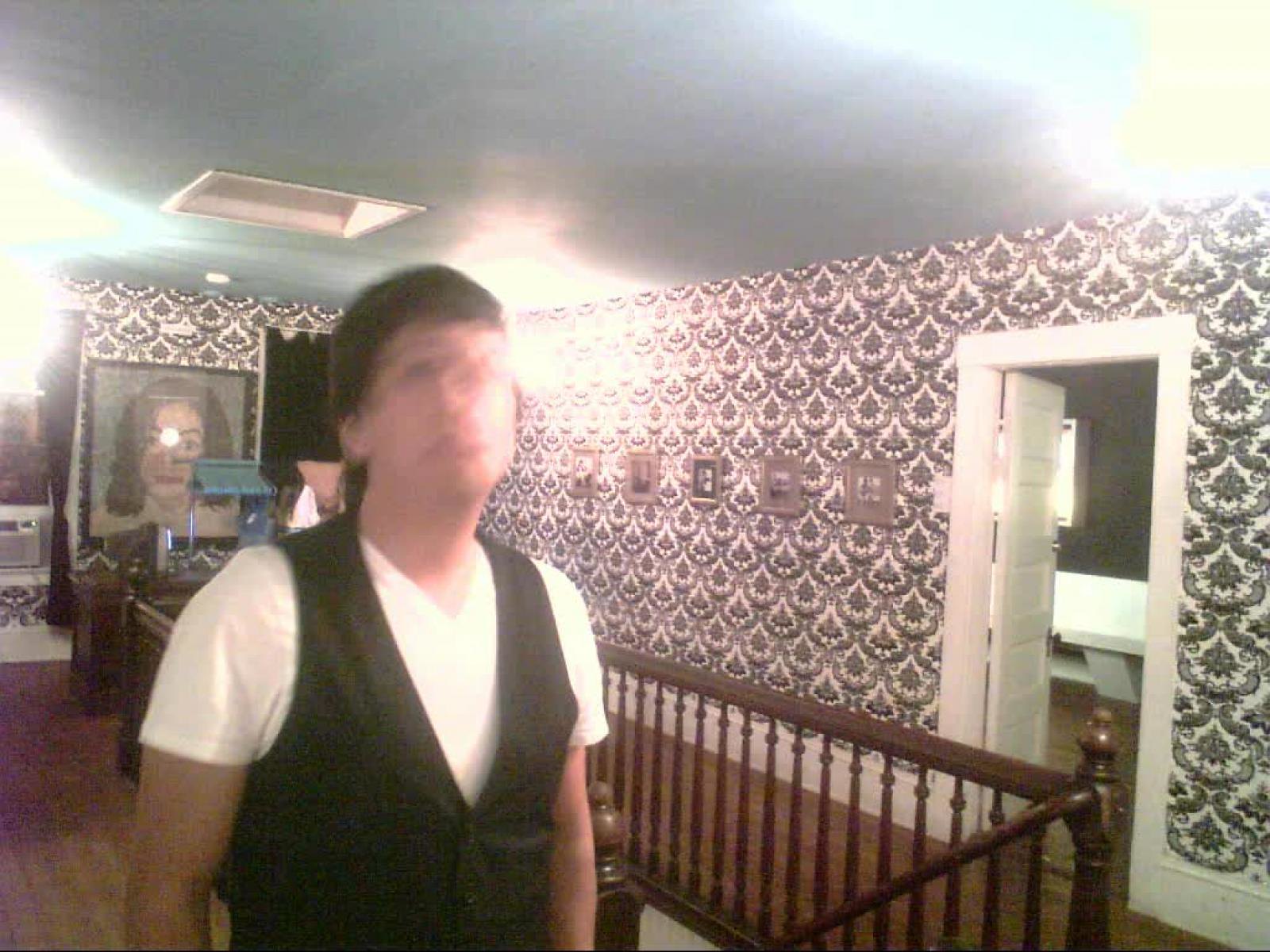The image captures a moment indoors, possibly at the top of a staircase in the upper level of a home. The main focus is a white male with short, dark brown hair, wearing a black vest over a white short-sleeved t-shirt with a V neckline. His face appears blurred, likely due to camera movement. He stands in a room with a reddish-brown short shag carpet and walls adorned with wallpaper featuring intricate, possibly floral designs in bluish or light greenish colors on a white background.

To the right of the image, there's an open white door leading into another room where a white bench is visible. Situated beside the door on the wall are five small square pictures, although their details are hard to discern. Behind the man, descending down, is a wooden banister of the staircase. A large square-shaped picture of Michael Jackson hangs prominently on the wall behind him. Some areas, especially on the ceiling, exhibit overexposed lighting, creating bright spots that obscure details, characterizing the vintage, somewhat gothic ambiance of the room.